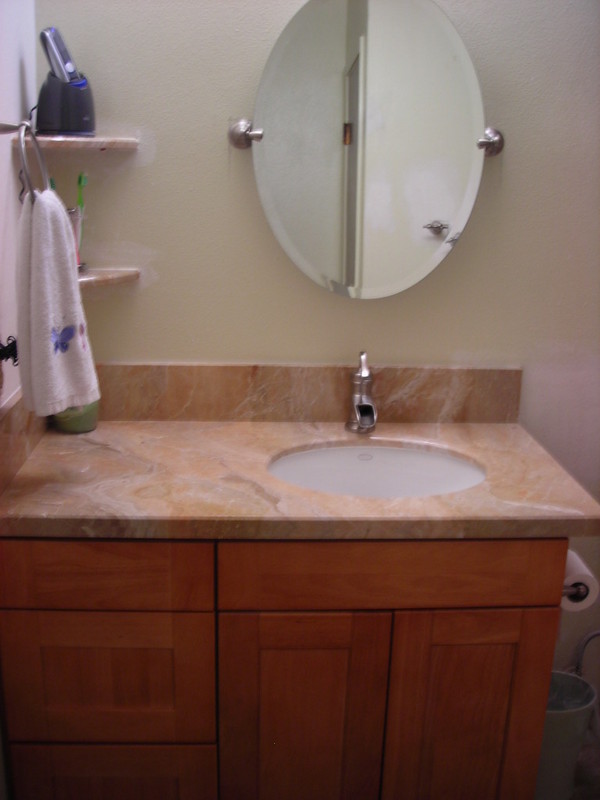This portrait-mode photograph captures the interior of a well-appointed bathroom. In the upper left-hand corner, there are two corner shelves. The top shelf holds what appears to be a charger, likely for an electric razor. On the lower shelf, a toothbrush holder is visible. Below these shelves, a silver towel holder is affixed to the wall. 

Prominently displayed in the top center of the image is an oval mirror. Through the reflection in the mirror, part of the bathroom door behind the photographer can be seen. Spanning from the left center to the right center of the image is a marbleized countertop with a sink and faucet. Beneath the countertop, wooden drawers and cabinet doors provide storage, with a toilet paper holder attached to the side of one of the cabinet doors. 

At the bottom of the frame, a blue pail, possibly used as a garbage can, rests on the floor. The image is rich in detail, offering a comprehensive view of the bathroom's various elements and layout.